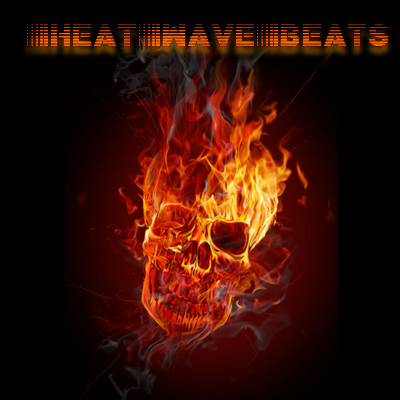This square image features a vividly detailed and centered flaming skull on a solid black background. The human skull, tilted slightly at approximately a 20-degree angle to the right, faces directly forward. The unique composition of the skull is depicted through flames, predominantly in hues of bright yellow, orange, and dark reddish tones, with a hint of blue swirling flames accentuating the fiery design. The eyes are dark voids, with the left eye showing faint flames while the right eye remains completely dark. Flames shoot dramatically from the nose and teeth, and burst intensely from the top of the skull, creating a red aura around the entire figure. Above the blazing skull, a line of heavily stylized, heat-distorted text in a bold gradient orange font reads "HEATWAVE BEATS". The energetic typography, with its fiery theme, seamlessly integrates with the graphic illustration, fading subtly at the top, adding to the overall intensity and visual impact of the artwork.